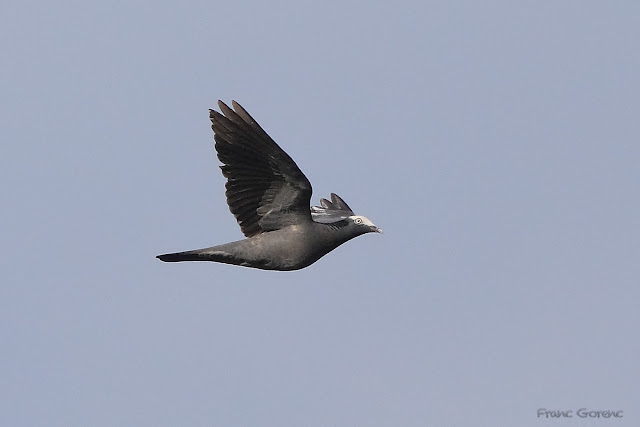In this painting, a bird in flight dominates a bluish-gray, periwinkle sky devoid of clouds or other elements. The bird, which resembles an eagle or crow, is seen from below, soaring slightly off-center to the left but primarily within the center of the image. With its wings raised above its body, the bird displays a straight tail and a dip in its belly. Its plumage features a spectrum of gray hues—dark gray, light gray—and the deepest shades mark its tail and feather tips. Notably, the bird's head and beak are white, as is one visible eye, which conveys a sense of fear. The bird's proportions suggest a moderate wingspan relative to its body size. In the bottom right corner of the painting, the artist's signature, "Frank Gorencic," underscores the realism of this artwork.